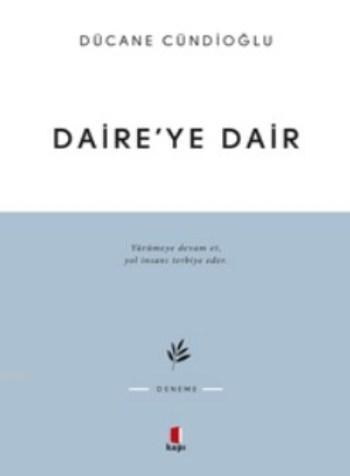The image shows a rectangular layout where the top half features a white background with two lines of text. The first line in black font reads "DUCANE CUNDIOGLU," while the second line, in larger, bolder black font, says "DAIRE'YE DAIR." Below this white section is a blue-gray square that contains detailed elements such as an illustration of a branch with five leaves, additional italicized text that is unreadable, two white lines flanking a black word, and at the very bottom, a red rectangle with black text beneath it. The overall image appears to be an advertisement in an unidentified language, possibly German, but its low resolution makes some elements difficult to discern.